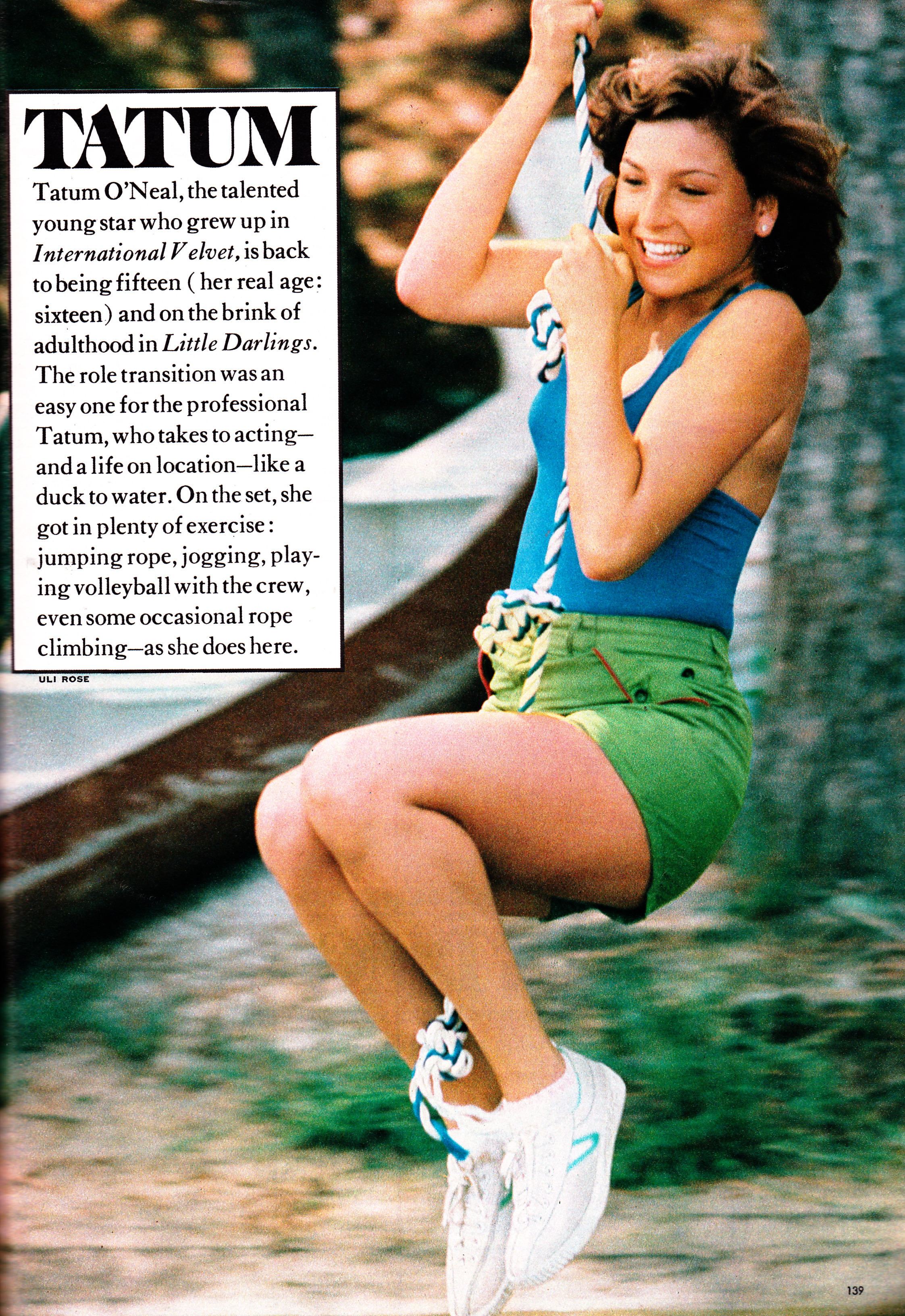This color photograph captures a young woman, likely Tatum O'Neal, joyfully swinging from a blue and white rope. The woman, who is a white female with short brown hair, is wearing a blue tank top, green shorts, and white sneakers. She clutches the rope with both hands, and her legs are curled upwards as she swings. A bright smile adorns her face, highlighting her youthful exuberance. The background features lush greenery, including several trees and a patch of grass, with a brown canoe visible among the foliage. The natural light suggests the photo was taken outdoors during daytime. In the upper left-hand corner, a black-bordered white text box prominently displays "Tatum" in bold. Below, the text elaborates on Tatum O'Neal's career, mentioning her transition back to her teenage years and her role in "Little Darlings." The text notes her various activities on set, such as jumping rope, jogging, playing volleyball, and rope climbing as showcased in this image. On the bottom right-hand corner is the black number "139." The photograph encapsulates a vibrant and active moment in the young star’s life.